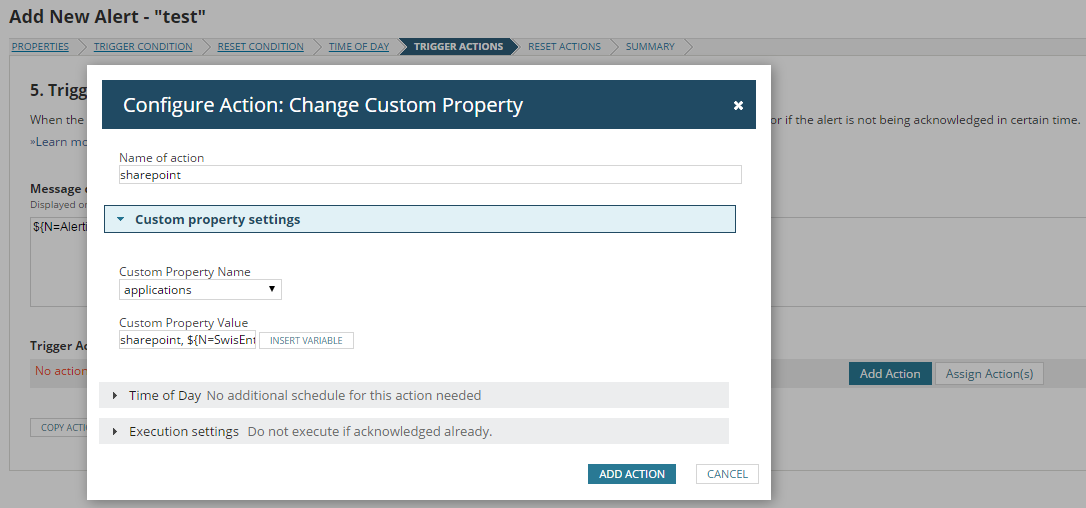This detailed screenshot captures the "Add a New Alert" interface, specifically on the "Trigger Actions" section. Prominently displayed at the top left is the header "Add New Alert" followed by "(Test)." The main menu, positioned horizontally at the top in blue, lists various categories: Properties, Trigger Condition, Reset Condition, Time of Day, Trigger Actions, Reset Actions, and Summary. 

The "Trigger Actions" category is currently active. A large white pop-up box labeled "Configure Action - Change Custom Property" is centered on the screen, with a close button (X) in the top right corner. Below this label, the box contains several fields and options in a white background. The first field, "Name of Action," has the text "SharePoint" entered. 

Further down is a section titled "Custom Property Settings," featuring a couple of dropdown boxes. The "Custom Property Name" dropdown is set to "Applications," while the "Custom Property Value" field shows "SharePoint" and "Code," with an adjacent button labeled "Insert Variable."

Two additional, non-expanded categories follow: "Time of Day," which specifies "No additional schedule for this action needed," and "Execution Settings," indicating "Do not execute if acknowledged already." 

At the very bottom right of the pop-up, there is a blue "Add Action" button and a white "Cancel" button, providing options to proceed or abort the operation.